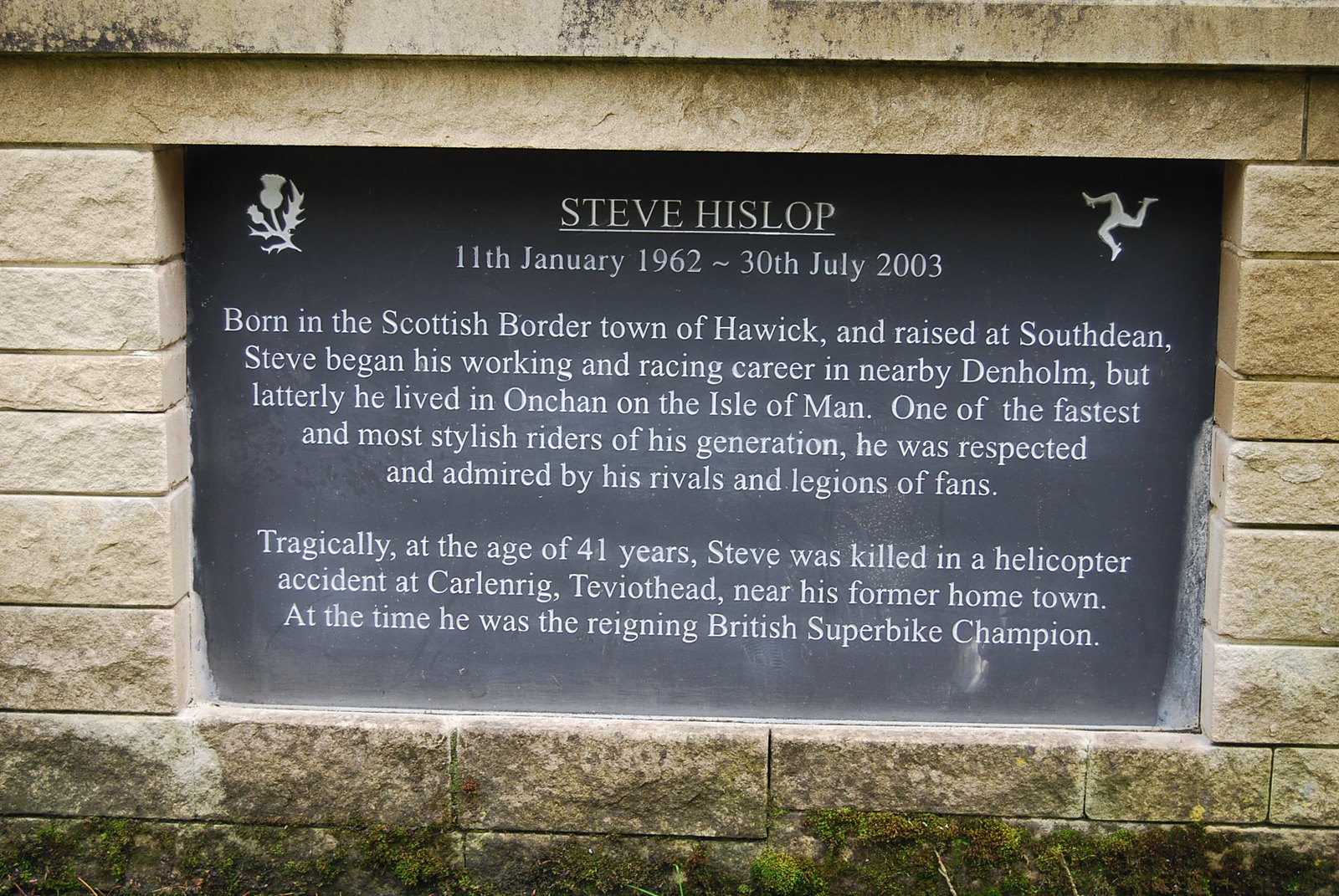The image depicts a memorial plaque inlaid within a structure made of layered brown stone bricks. The plaque itself is black with engraved white text and is placed in the middle of a stone setting, which is darker and appears to have moss at the base. At the top left of the plaque is a white silhouette of a flower with a hanging leaf, and to the top right is an abstract depiction of three feet arranged in a triangular pattern. The plaque commemorates Steve Hislop, whose name is prominently underlined at the top. Below his name, the dates "11th January 1962 to 30th July 2003" are inscribed. Further text reads: "Born in the Scottish border town of Hawick and raised in South Dean, Steve began his working and racing career in nearby Denholm but laterally he lived in Onchan on the Isle of Man. One of the fastest and most stylish riders of his generation, he was respected and admired by his rivals and legions of fans. Tragically, at the age of 41, Steve was killed in a helicopter accident at Carlingrig, Teviot Head, near his former hometown. At the time, he was the reigning British Superbike champion." The plaque and stones around it form a solemn tribute to the late racer, set against a background of rustic, darkened stone and natural elements.